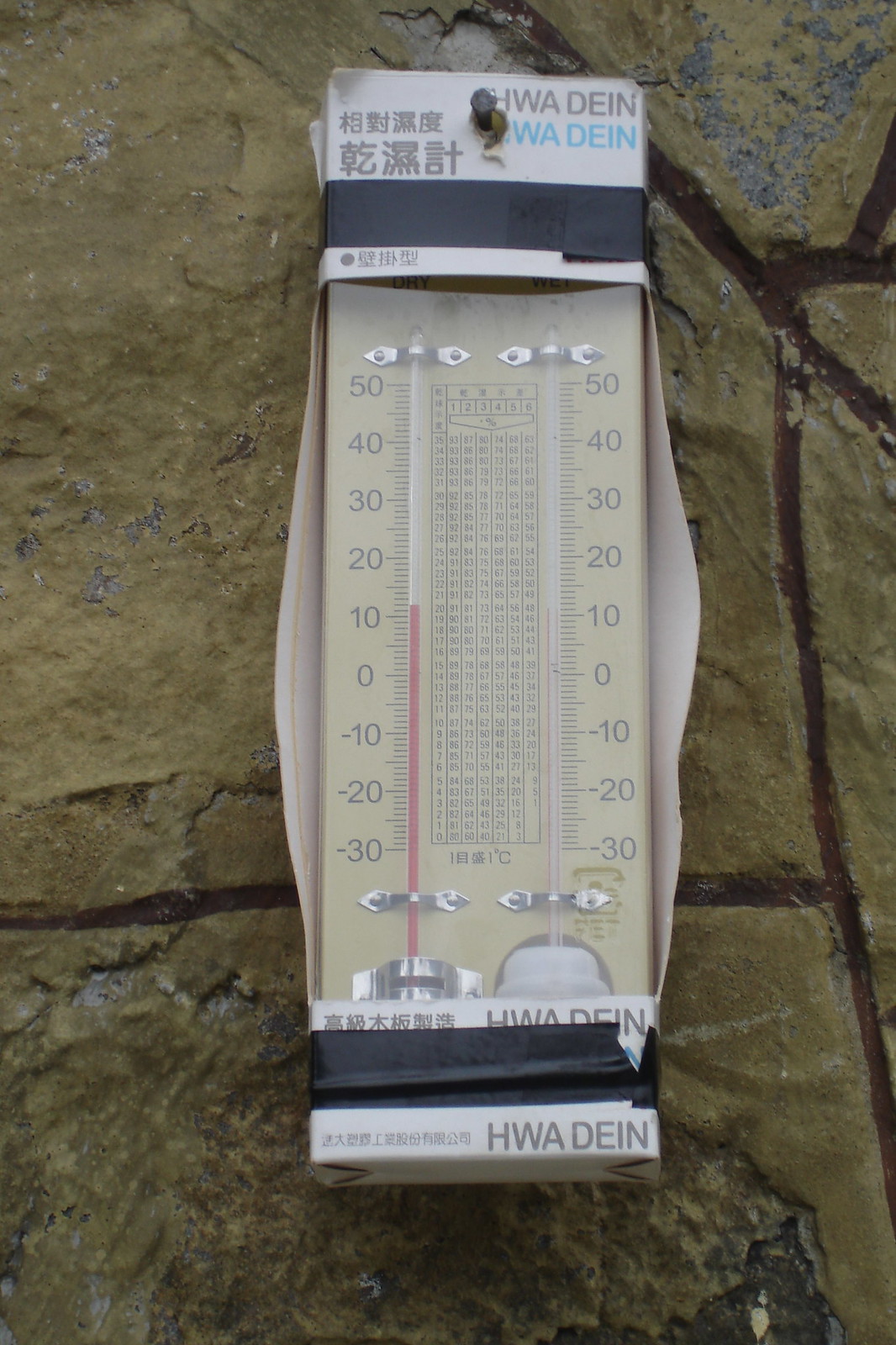The image depicts a boxed thermometer mounted on a stone or tile floor. The flooring features a combination of brown, gray, and black tiles interspersed with brown grout lines. The thermometer is enclosed in a box with Asian lettering and displays the text "IWA DEIN" twice; once in black font at the top right corner, and directly below it in blue font. A nail secures the box to the wall, and there is a black strip of tape beneath the nail.

The thermometer box contains two thermometers, both with a measurement range from -30 to 50 degrees. The left thermometer currently reads just over 10 degrees. Below the thermometers, another white section of the box features the text "HWA DEIN," accompanied by an additional black strip of tape.